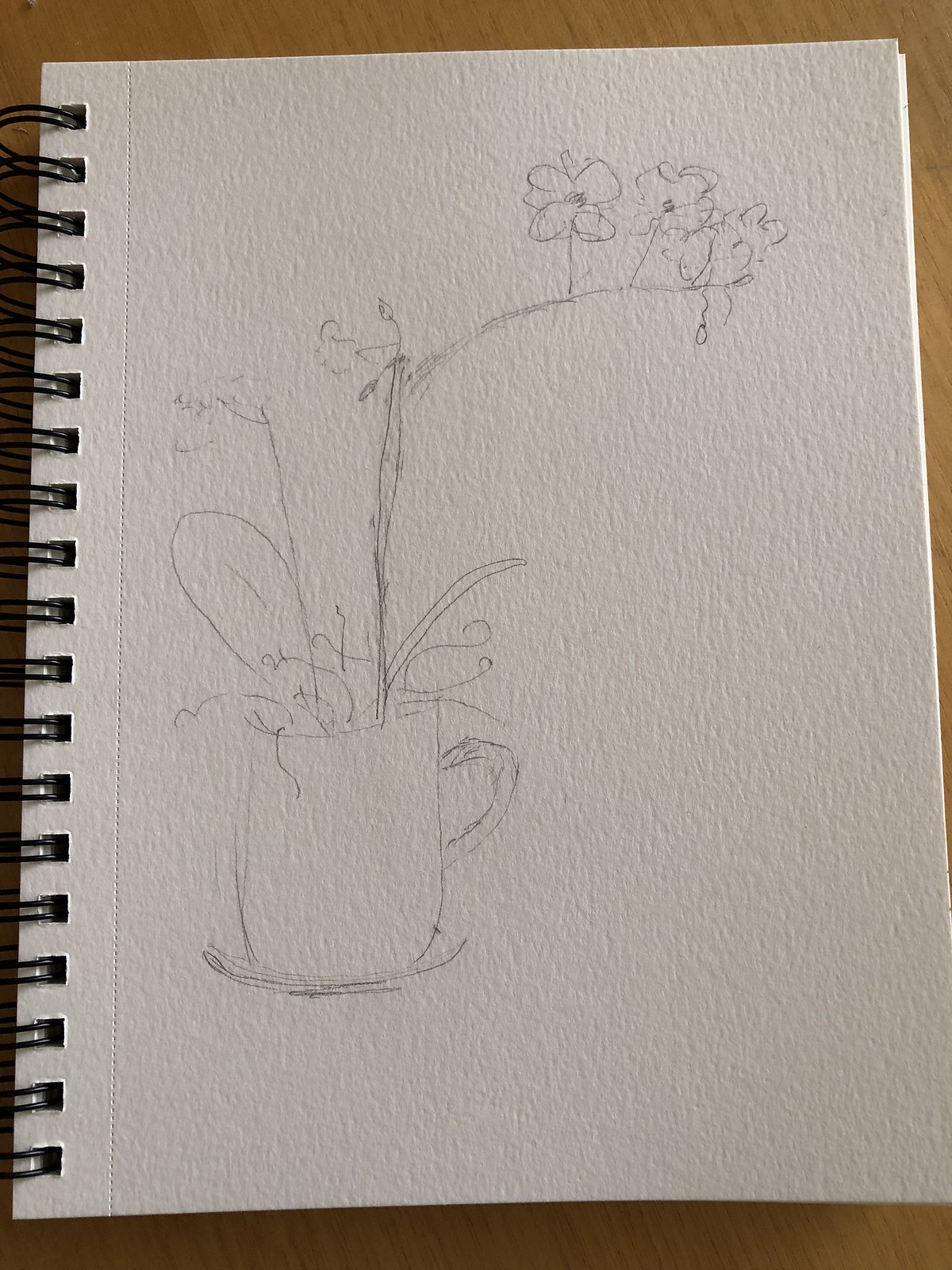This image features the cover of a white, textured, spiral-bound sketchbook, resting on a brown, wood-grain tabletop. The notebook's black metal spiral binding runs along the left edge, and the cover appears to have a serrated edge, hinting at perforated pages inside for easy removal. The lightly drawn pencil sketch on the cover depicts a basic outline of a coffee mug with a handle on the right side. The mug, which resembles both a tea and coffee cup, sits on what seems to be a bowl or plate. Emerging from the mug are various plant elements, including leaves and flowers. A long stem extends to the right side of the sketch, adorned with flowers, while additional leaves can be seen on the left.